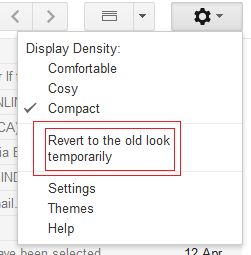The image is a square screenshot capturing a pop-up message overlaying another message in the background. The background message, partially visible at the top left and right, includes a navigation bar with icons. On the upper left are back and forward arrows, followed by a rectangular icon with three lines, the function of which is unclear. This is followed by a drop-down menu. The upper right corner of the background message shows a black settings icon with its own drop-down menu.

On the left side, the background message lists multiple items in rows numbered from 1 to 9, with more extending beyond the visible area. Each row starts with partial text fragments such as "if," "li," "ca," "ia," "ind," and "ail."

The pop-up message, which stands out with a white background compared to the grayish tone of the background message, begins with the options for "Display Density" listed as "Comfortable," "Cozy," and "Compact," with a checkmark next to "Compact." 

Additionally, the pop-up message features two red outlined rectangles around an option labeled "Revert to the old look temporarily." Below this, there are options for "Settings," "Themes," and "Help."